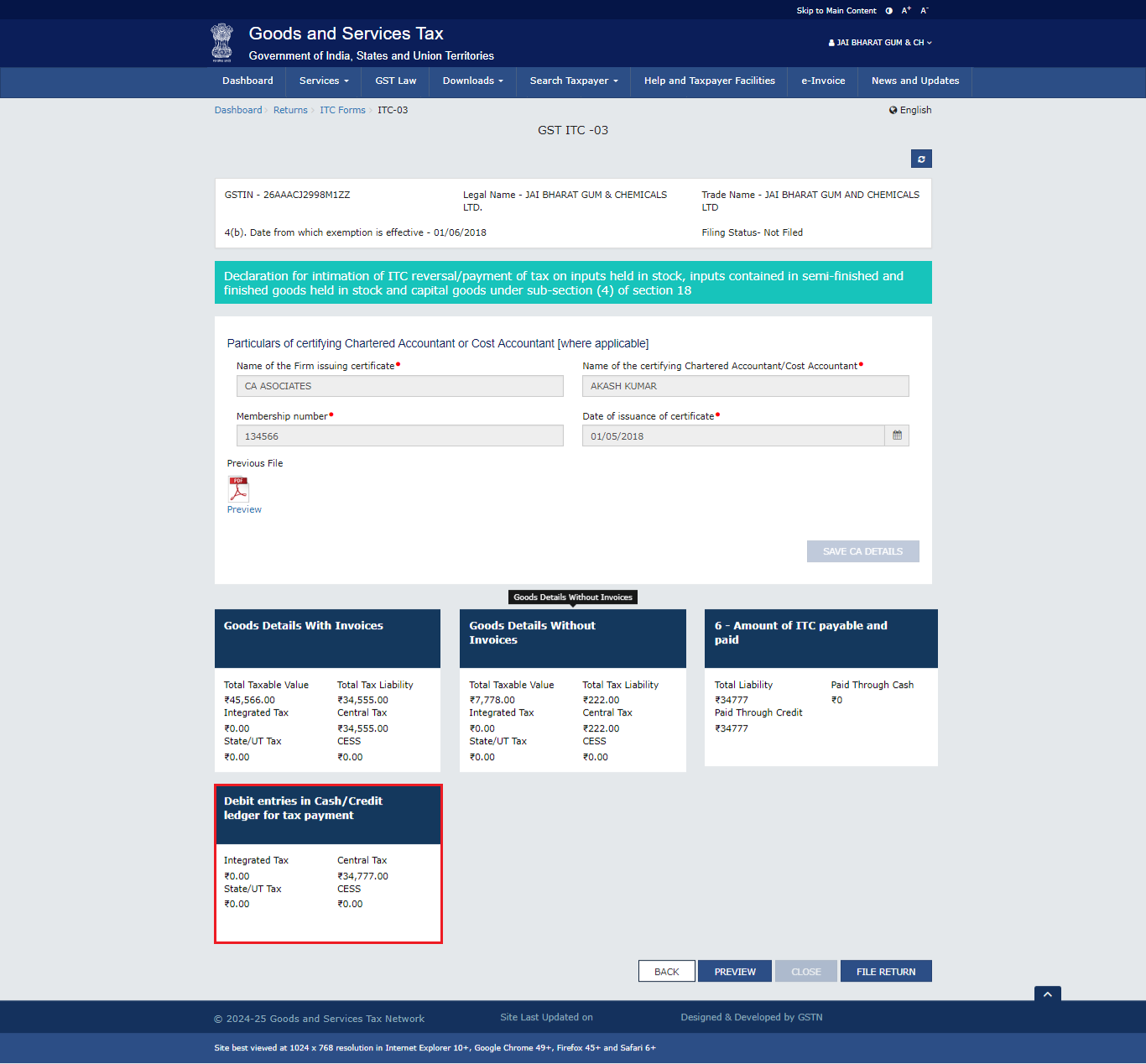The image features a structured dashboard interface related to GST (Goods and Services Tax) management. At the very top, a dark blue banner prominently displays the text "Goods and Services Tax" in white. Directly beneath this, another blue rectangle contains navigation options labeled: Dashboard, Sessions, and Search.

Below the navigation bar, there's a section labeled "O-S-T-I-T-C-03" at the top. Adjacent to it, a small green box with white text reads "Deactivation", followed by two lines of very small, unreadable white text.

The main interface is divided into four long rectangular sections, each with a gray background and placeholder text. Beneath these sections, four distinct categories are displayed in box format: 
1. **Details**
2. **Goods Details with Invoices and Goods Details without Invoices**
3. **Amount of TTC Payable and Paid**

A distinctive box outlined in red is labeled "Cash Credit for Tax Payment" to highlight its importance. Finally, at the bottom of the interface, there's a blue button labeled "File Return," indicating the action users should take.